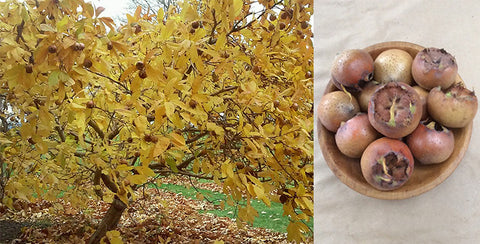The image is a split-screen composition featuring two distinct yet related photographs. On the right, a wooden bowl sits on an off-white, possibly textured surface, containing a collection of round fruits in varying shades of reddish-brown and lighter tones. Some of the fruits appear to be rotted or damaged, with visible jagged cuts exposing their inner flesh adorned with greenish lines. On the left, a short tree with a thick, dark brown trunk and branches is depicted, its yellow, golden-hued leaves contrasting against the gray, sunless sky. The tree bears the same type of brownish fruit seen in the bowl. The ground beneath the tree is strewn with fallen leaves, interspersed with patches of green grass.